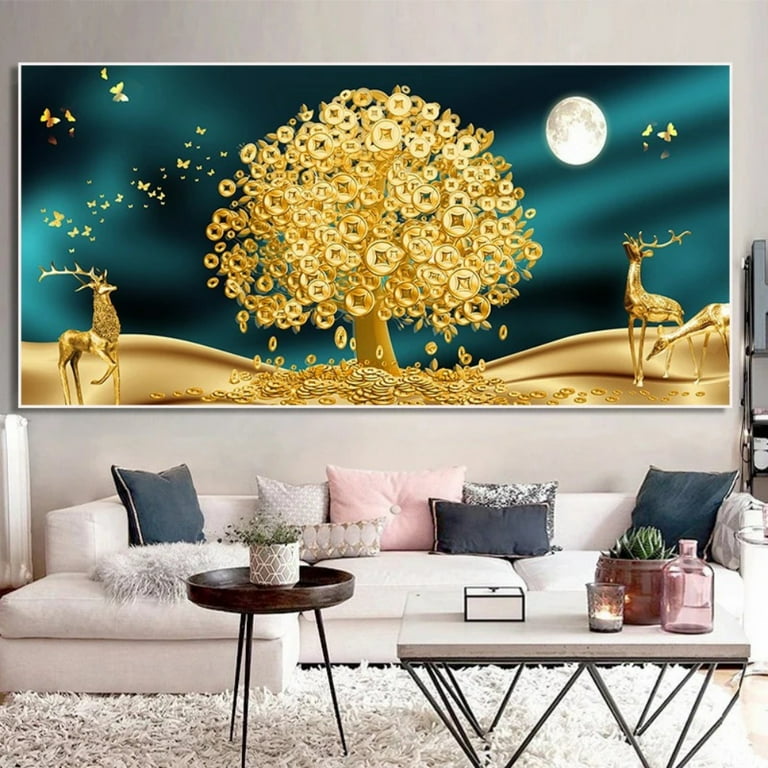This detailed image showcases a beautifully decorated living room highlighted by a prominent wall ornament. The centerpiece of the room is a white couch, adorned with an array of pillows in shades of blue, white, gray, and pink. Underneath the couch lies a large fur rug, adding a touch of luxury and comfort. 

Behind the couch, a captivating wall picture features a majestic gold tree, with gold coins instead of leaves cascading down into a pile at its base. Flanking this tree are three golden deer, their antlers gracefully extending upwards. Gold butterflies are scattered around the scene, set against a backdrop of golden hills, a blue sky, and a large, luminous white moon.

In front of the couch, a white coffee table with black metal legs holds two plants, several boxes, and a few candles. Adjacent to it is a smaller, round wooden table with three metal legs, further enhancing the room's elegant aesthetic.